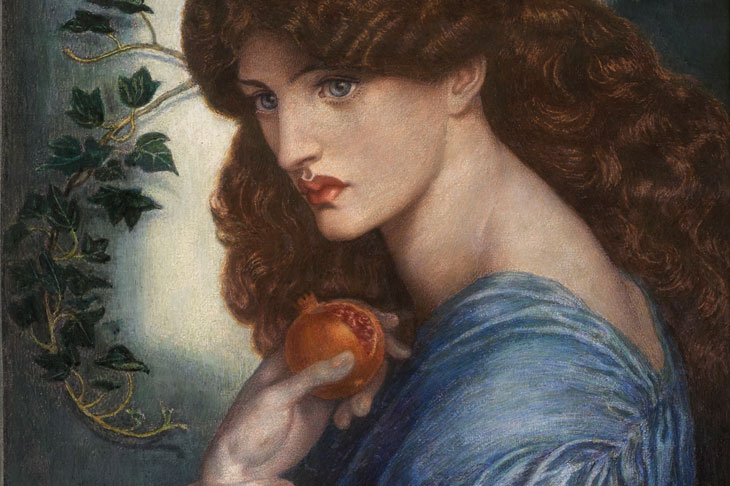This detailed painting depicts a young woman from her shoulders up to her forehead, with the very top of her head cut off. She is wearing a blue dress that has a low-cut back, exposing some skin before the material begins again over her shoulders. The woman has long, wavy brown hair cascading down past her shoulders. Her bright blue eyes and red lips, possibly enhanced with lipstick, stand out vividly against her fair skin. She is gazing off to the left, with her left hand raised near her chin, delicately holding a fruit. The fruit appears to be an orange or possibly a peach, characterized by its orange exterior and similarly colored interior, with a small crown-like element on top. In the background, there is a white wall adorned with a vine-like branch with leaves sprawling mostly on the left side of the image. The lighting behind her head creates a subtle halo effect, while the rest of the wall appears dark, adding depth and contrast to the classic 17th or 18th-century style of the painting.